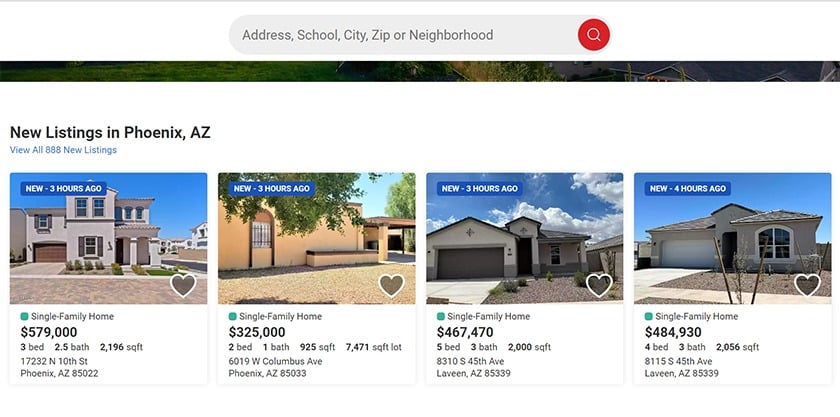The image depicts a housing website showcasing available properties for sale. At the top of the interface, there's a search bar allowing users to input criteria such as the address, school, city, zip code, or neighborhood to refine their property search. The highlighted section features new listings in Phoenix, Arizona, and a clickable option to view all 888 new listings.

The displayed segment showcases four single-family homes with detailed information:

1. The most expensive property listed at $579,000 features three bedrooms, two and a half bathrooms, and spans almost 2,200 square feet. The specific address is provided.

2. The least expensive property, priced at $325,000, includes two bedrooms, one bathroom, and is 925 square feet. The lot size is 7,471 square feet, and the address is listed.

3. Another home available for $467,000 offers five bedrooms and three bathrooms.

4. The final property is priced at $484,000, featuring four bedrooms and three bathrooms, and is nearly 2,000 square feet.

All the properties listed include images and indications of their recent postings, marked as "new three hours ago" or "new four hours ago".